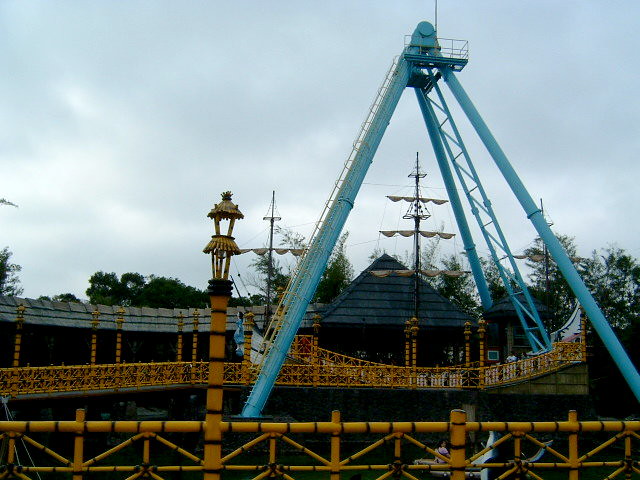In this vibrant and detailed image of an apparent amusement park taken during the day, we start with the foreground, dominated by a prominent yellow and black fence that runs horizontally across the bottom of the scene, wrapping around to the left. Noteworthy are its alternating post colors, suggesting caution, and various elements, including lamp posts with dual covers. Just behind the fence, the scene extends into a walkway bordered by this colorful barrier, leading centrally towards a strikingly tall blue tower.

This blue tower, supported on all sides, features a ladder ascending to a viewing stand enclosed by railings. Adjacent to this, another taller, circular safety ladder reaches upwards. In the middle ground, a yellow and black striped post rises, equipped with a light on top, augmenting the scene's industrial aesthetics. Beside this post, a unique structure resembling a blue pyramid with four posts converges upward, topped with a ladder, contributing to the elaborate framework of the setting.

Further back, a wooden A-frame roof house, with a bluish-gray tone, appears nestled amidst large green trees towering above all structures, highlighting the grand scale of the amusement park’s environment. Enhancing the historical and public setting ambiance, a mast equipped with three furled sails stands in front of the building. The entire scene is capped by a densely cloud-filled sky, presenting a dynamic contrast between the blue, gray, white, and green elements throughout the image.